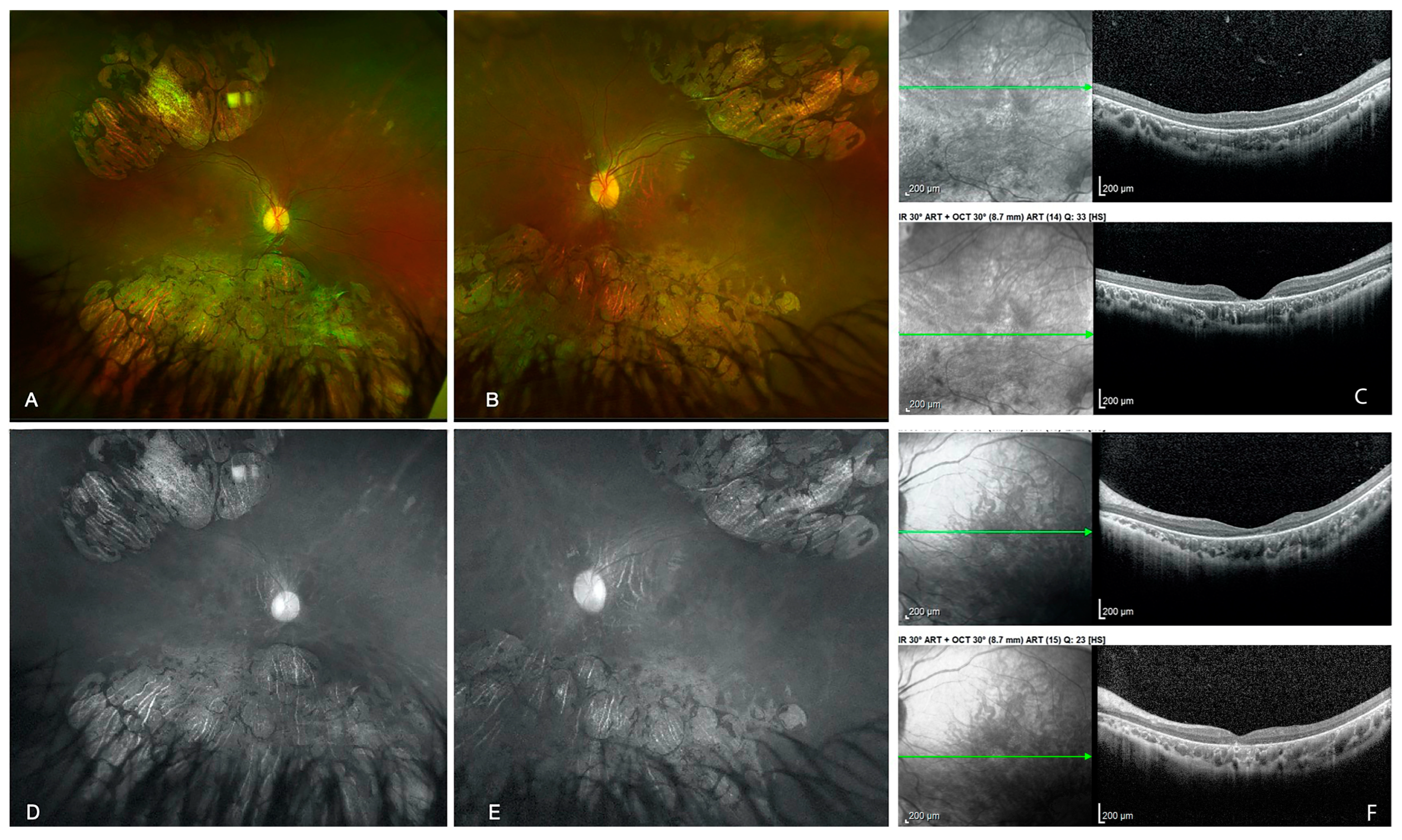This image appears to be a detailed medical slide, likely part of a scientific publication, showcasing a series of diagnostic photographs of a human eye. The layout is divided into multiple sections with various close-up images and graphs. On the left side, there are four labeled boxes: A, B, D, and E. Boxes A and B are colorized, displaying abstract patterns in rusty browns with a distinct white round object, likely an eye with visible blood veins and tissue growths. Boxes D and E are the black and white versions of A and B, providing a clearer yet less detailed view of the same structures.

To the right, additional boxes are arranged, with four in black and white depicting a fleshy line-shaped structure. These images are likely cross-sectional views or different angles of the eye, highlighting its internal components and veins. Further labels, such as C and F, suggest these images were taken from different perspectives or using different photographic techniques. Accompanying these visuals are scientific annotations indicating measurements and methodologies, such as "IR-30 ART plus OCT-30." One particular graph with a green arrow points to a 200-micrometer scale, potentially measuring wavelength or another scientific variable related to eye structure or function.